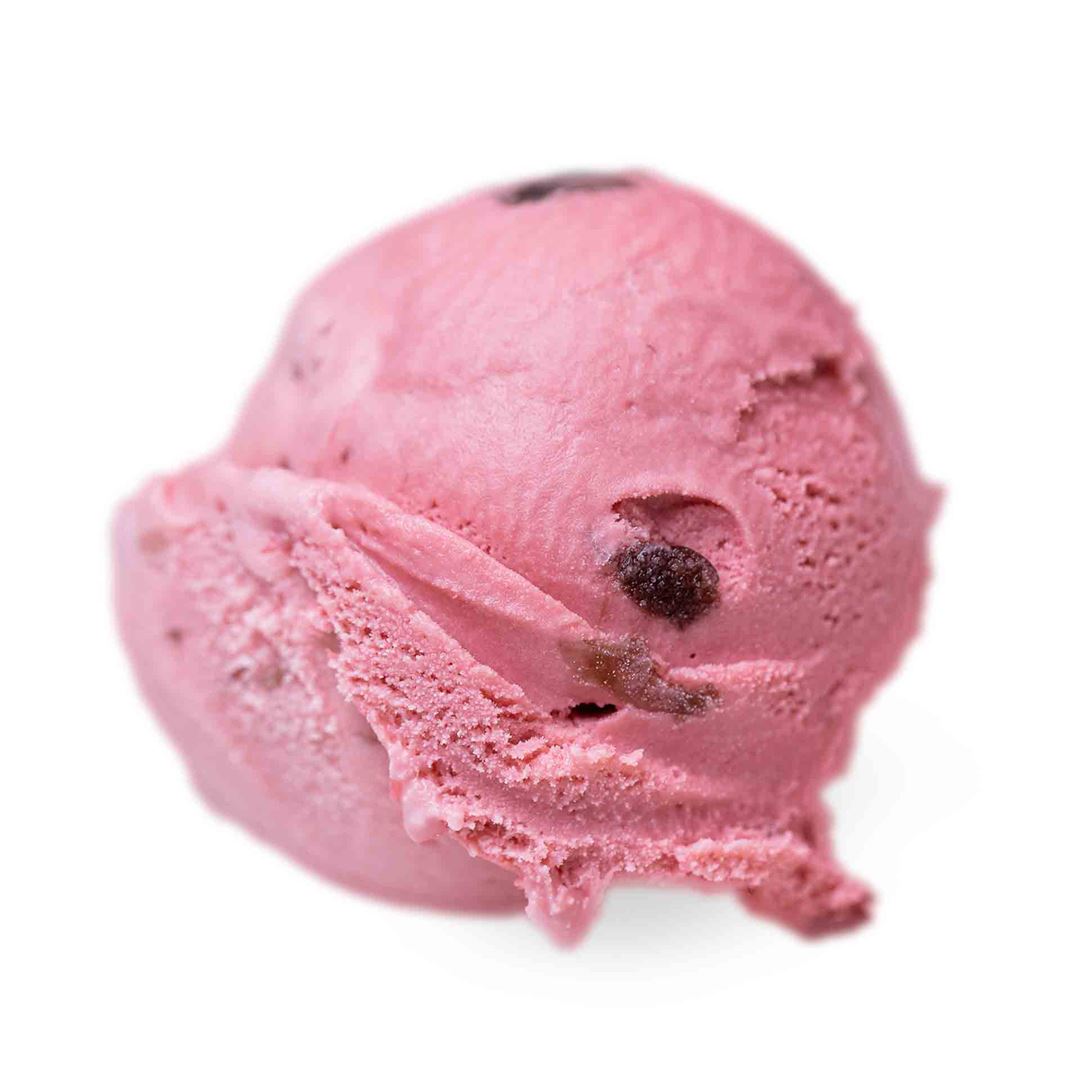In this close-up photo, a single scoop of ice cream is set against a white background. The ice cream is predominantly bubblegum pink with various shades and textures that create a visually captivating image. The focal point includes a roughly textured surface with ice crystals scattered across it. Notably, there are black dots and darker maroon splotches that resemble pieces of fresh fruit, potentially strawberry, as the red splotches and seed-like specks throughout the ice cream suggest. The left side of the scoop transitions into a lighter pink color, which becomes blurred, adding depth to the image. The ice cream's wavy texture indicates the scoop's origin, and the overall well-lit setting highlights its vibrant color and intricate details.